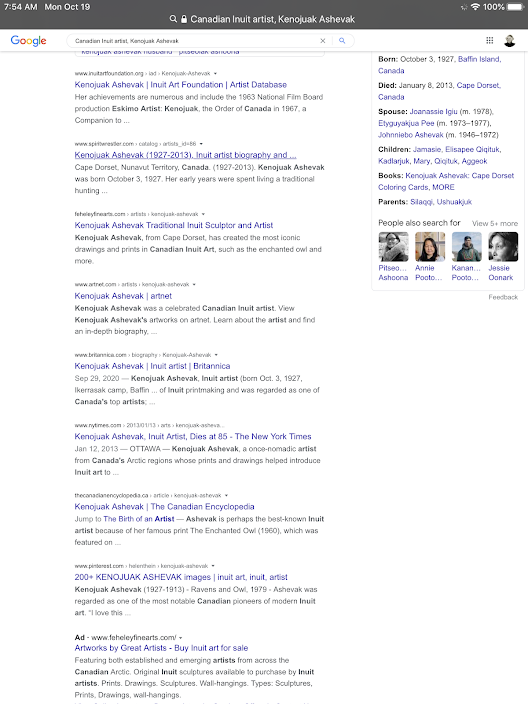A screenshot of a Google search results page is displayed on a mobile device. The image captures the screen at 7:54 a.m. on Monday, October 19th. The status bar at the top shows a full Wi-Fi signal and a battery life of 100%, indicated by the battery icon. Beneath the status bar, the lock icon signifies a secure connection in the search bar.

The search query entered pertains to Kinojuak Ashevak, an esteemed Canadian Inuit artist. The Google logo, adorned in its signature colors of blue, red, yellow, and green, sits prominently above the search results. To the far right of the screen, a selection of photos associated with the artist appears.

The search information reveals that Kinojuak Ashevak was born on October 3rd, 1927, in Baffin Island, Canada, and passed away on January 8th, 2013, in Cape Dorset, Canada. The results also note the artist's personal details, including having had three spouses, and list their children with clickable hyperlinks for further information. Additionally, several of the artist's books and their parents are mentioned, showcasing the breadth of Ashevak's creative and familial life.